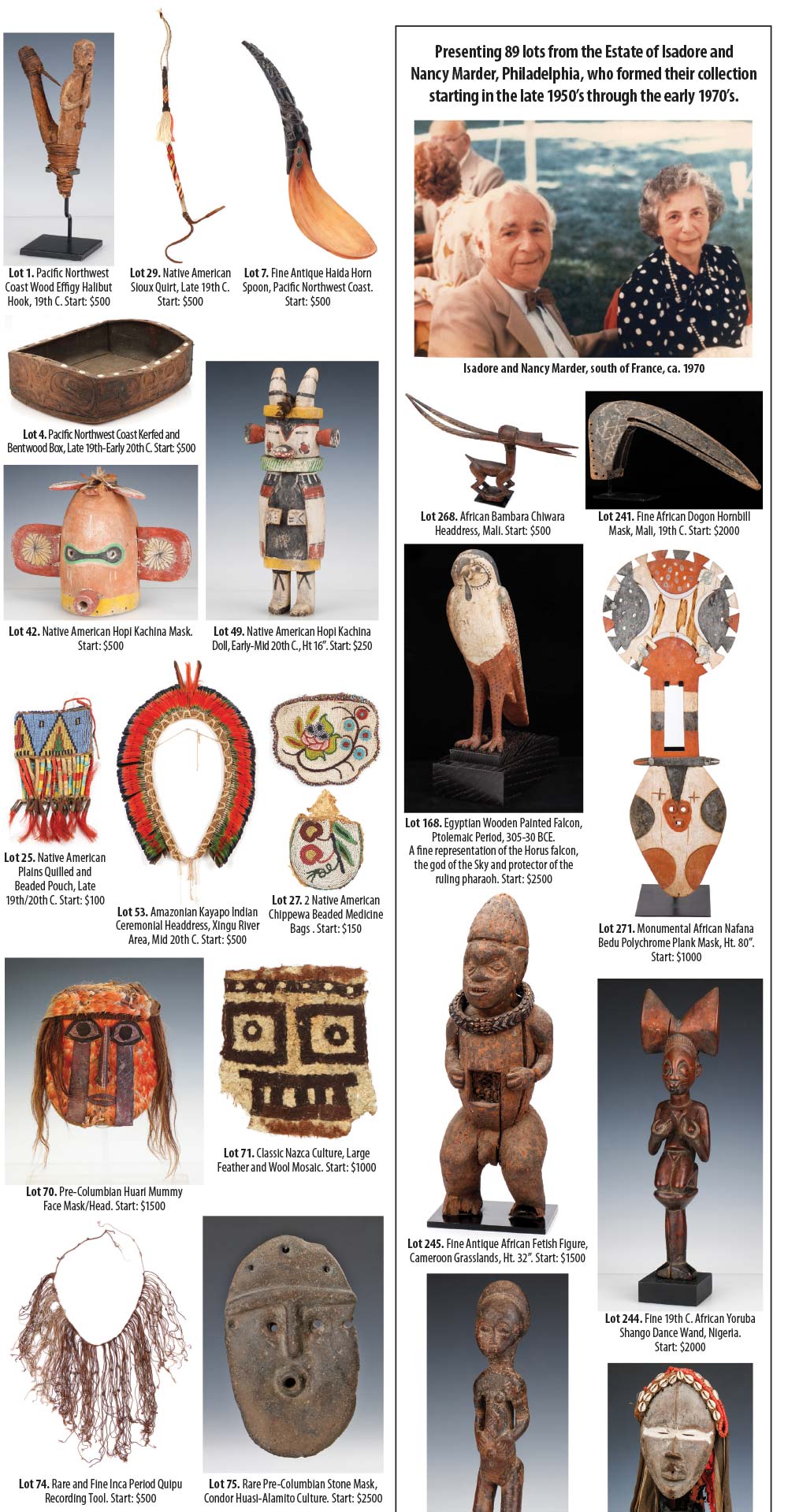This image is a detailed brochure spanning two pages, highlighting an auction of 89 lots from the estate of Isidore and Nancy Martyr of Philadelphia. The collection, amassed from the late 1950s through the early 1970s, features a variety of artifacts including statues, masks, and jewelry. The right page prominently displays black text above a photo of Isidore and Nancy taken in the south of France in 1970, with Isidore in a brown suit and gray hair, and Nancy in a black polka-dotted shirt. The artifacts, many of which are African, Egyptian, and Native American, are meticulously described and priced beneath their images. Examples of the items include a Lot 1 Pacific Northwest Coast Wood Epogee Halibut Hook and Lot 29 Native American Sioux Court from the late 19th century starting at $500.